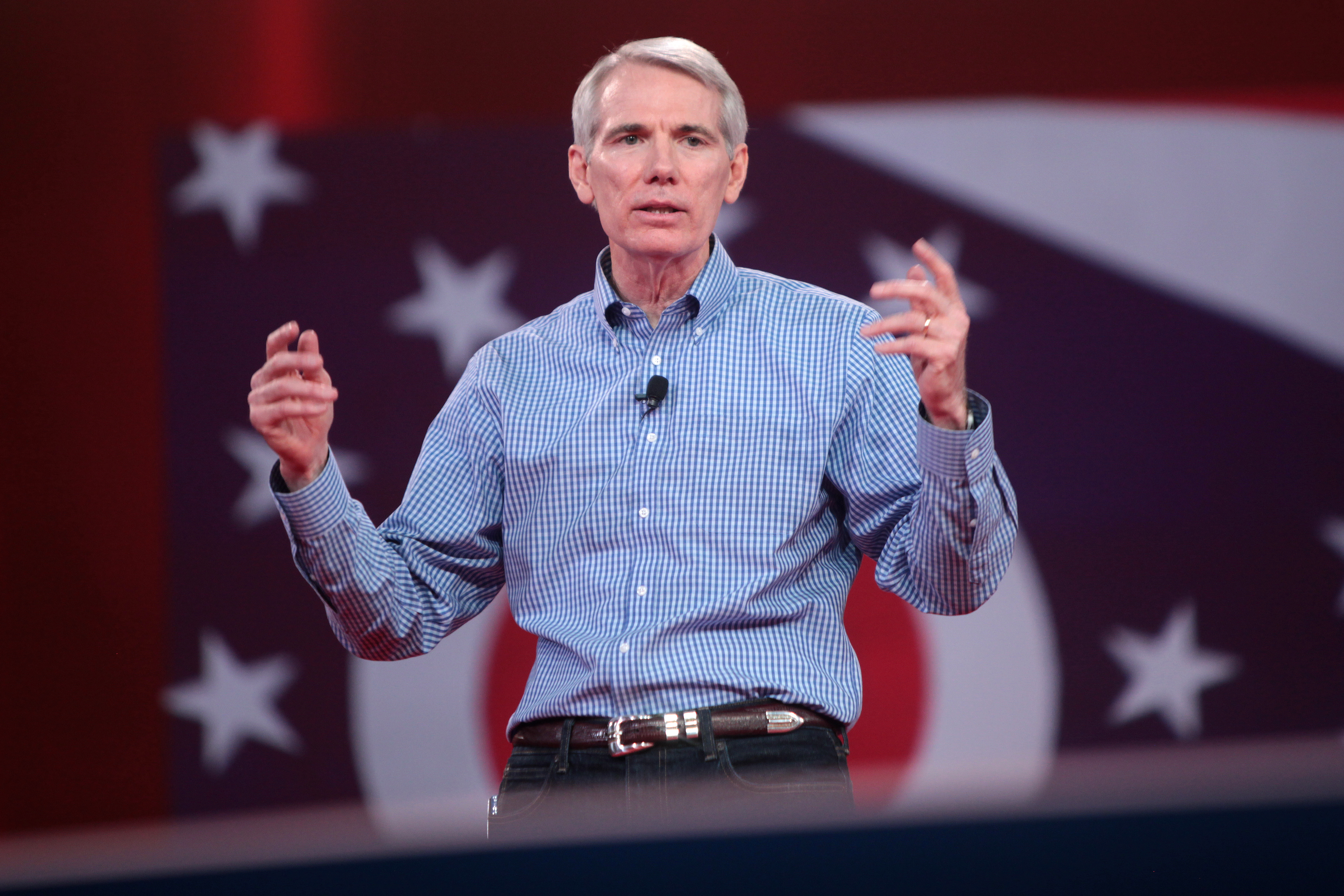The photograph features a gray-haired man with his hair parted to the side, standing on a stage. He is dressed in a light blue and dark blue shirt, adorned with white buttons and a black microphone clipped just below the collar. He wears blue jeans secured with a brown belt featuring a silver buckle, and his arms are bent at the elbows, raised to shoulder height on either side of him. He also sports a wristwatch and a wedding ring on his left hand. Behind him, there's a stylized backdrop resembling the American flag, showcasing red, white, and blue elements, with visible white stars and stripes. The setting suggests he might be addressing an audience, possibly in a formal or public speaking context.